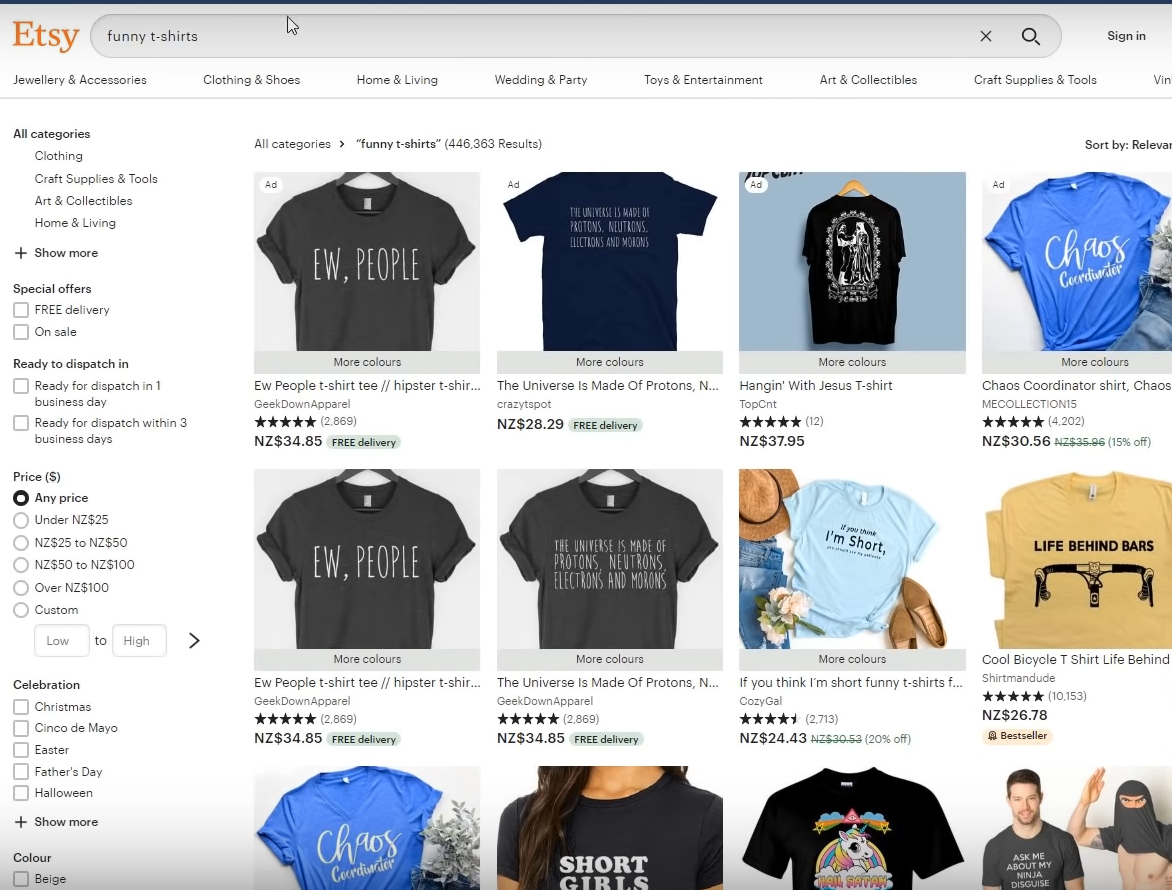Here is a detailed and refined caption for the described screenshot of an Etsy page:

---

The screenshot displays an Etsy webpage showcasing a search for "funny t-shirts." The recognizable orange Etsy logo is positioned at the top left corner of the page. Directly to the right of the logo is an elongated search bar, containing the text "funny t-shirts." Adjacent to the search bar on the far right are the "X" button for clearing the search input and the magnifying glass icon as a search button. Further right, there's a prominent "Sign In" button.

Below the search bar is a top navigation menu featuring various shopping categories: Jewelry & Accessories, Clothing & Shoes, Home & Living, Wedding & Party, Toys & Entertainment, Art & Collectibles, and Craft Supplies & Tools.

On the left side of the page, a sidebar with multiple category options is visible. At the top of the sidebar, it reads "All Categories", followed by sections labeled "Special Offers", "Ready to Dispatch", "Price", "Celebration", and "Color". Under the "All Categories" section, subcategories include Clothing, Craft Supplies & Tools, Art & Collectibles, Home & Living, and an expandable link indicated by "Show More".

In the "Special Offers" section, options such as "Free Delivery" and "On Sale" are indicated by checkboxes. The "Ready to Dispatch" category contains two additional checkboxes. Under the "Price" section, there are six radio buttons for different price ranges, followed by input fields for specifying price from low to high.

---

This caption provides a clear and comprehensive description of the Etsy webpage layout and its various components.